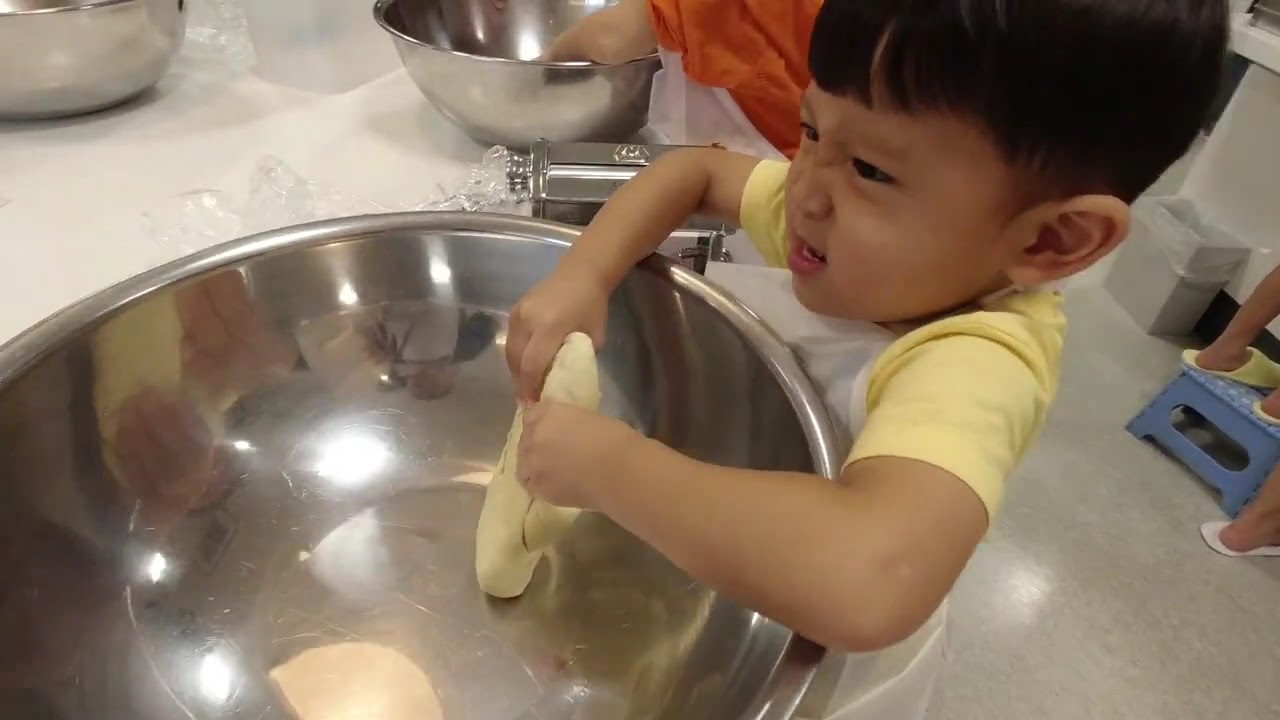This is a high-definition, landscape-oriented color photograph capturing a charming and lively scene of a young Asian boy, around three to four years old, deeply engaged in an activity at what appears to be a kitchen counter. The boy, who has dark hair and dark skin, is standing on a tiled kitchen floor, wearing a bright yellow shirt. Positioned towards the right side of the image, he faces left, concentrating intently on a large stainless steel bowl in front of him. With a playful grimace, he has his hand submerged in the bowl, playing with an irregularly shaped piece of beige dough. 

Next to him, a partially visible person in a red, yellow, or orange top—likely his mother—is also engaged with a similar, smaller stainless steel bowl. This person’s upper body and hands are visible, suggesting close interaction, possibly guiding or accompanying the boy in the dough-making task. Between them on the counter, various kitchen items, including what seems to be a stainless steel pasta machine, add to the bustling kitchen atmosphere. Various other bowls and utensils are scattered around, hinting at a busy, perhaps educational or family-centered cooking session occurring in the midst of the day. 

The vivid colors of silver, yellow, red, white, and beige highlight the photo’s realism, emphasizing the textured and tactile nature of the cooking materials and the human expressions in the scene.